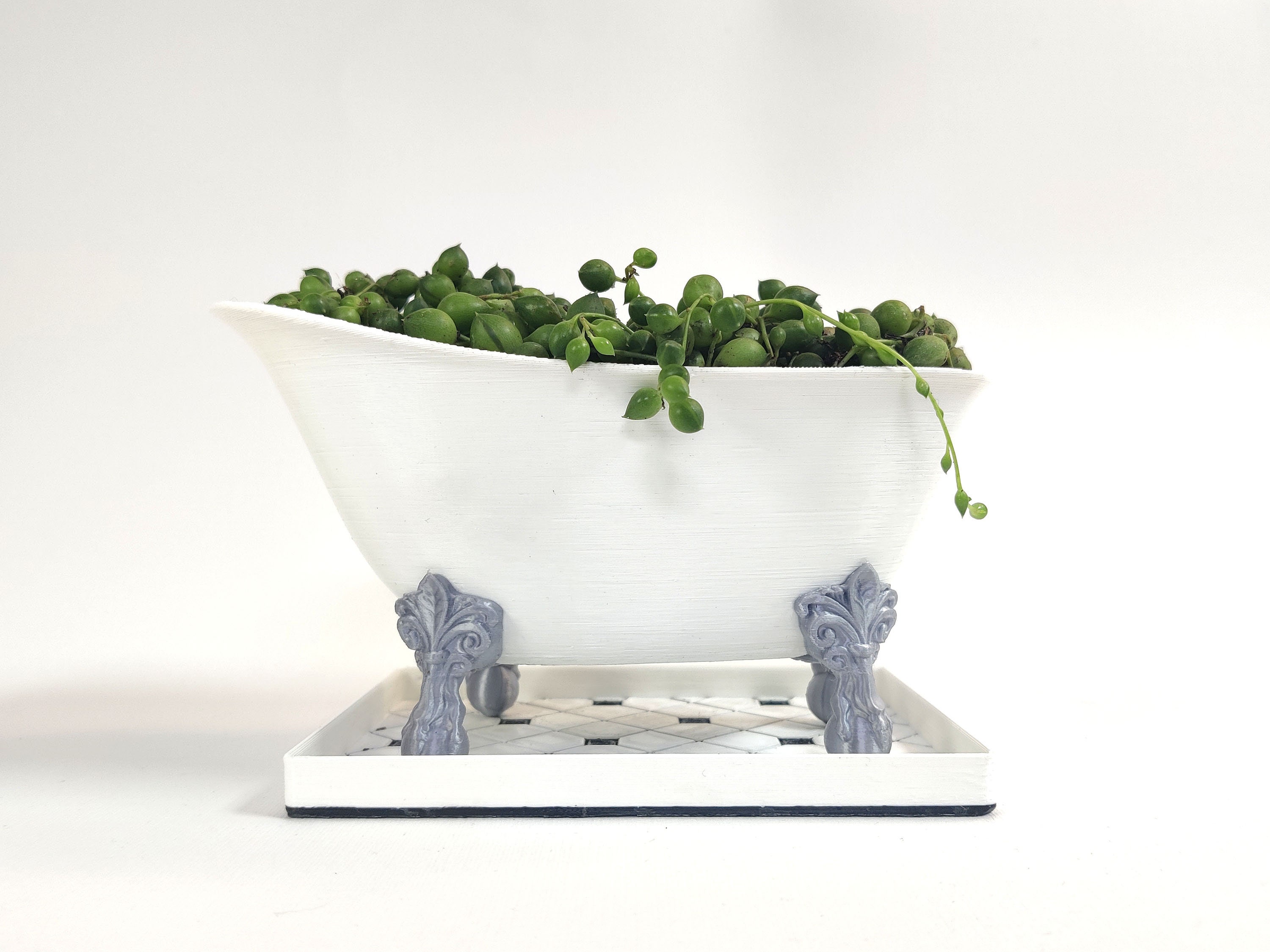This photograph features a charming, old-fashioned, ceramic bathtub-shaped dish, which adds a whimsical touch to the scene. The dish is held up by four ornate legs with a fleur-de-lis design at the top of each, and the legs are a shade of pale blue or grey. The bathtub itself is white with a subtle horizontal stripe pattern in very light grey. 

Inside the tub is a lush plant consisting of shiny, deep green leaves and bulbs that resemble peas, likely a rosary plant, attached to thin, pale green stems. One of these stems is gracefully draping over the right side of the dish, adorned with small green buds. 

The bathtub is placed on a white, square dish featuring a striking black and white crisscross or geometric square pattern on the top surface. The pure white background contrasts sharply with the intricate design of the dish and the vibrant greenery of the plant, creating a visually appealing and detailed composition.